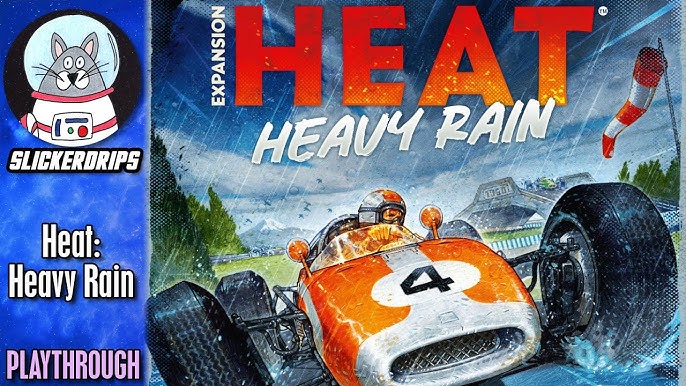This image is a detailed scan of an advertisement likely for a game expansion. It prominently features a cartoon-style drawing of a race car driver in an orange boxcar-style vehicle with oversized tires protruding from the body, connected by arms. The car, adorned with a numeral 4 on its front and a small windshield, is shown racing on a track in heavy rain. The driver, wearing a white helmet with an orange stripe and orange goggles, peeks above the windshield as he races forward. The background depicts a stadium and an orange-and-white striped windsock flapping in the storm. At the top of the image, the large word "HEAT" in orange is followed by the smaller white text "HEAVY RAIN." To the left edge of the picture, a vertical blue strip contains additional information and an illustration of a gray cat in a fishbowl helmet and white astronaut outfit, labeled "Slicker Drips." This strip also includes the text "Heat Heavy Rain" and "Purple Playthrough." The overall composition blends vibrant colors and dynamic elements, reflecting the intensity and excitement of the race in adverse weather conditions.